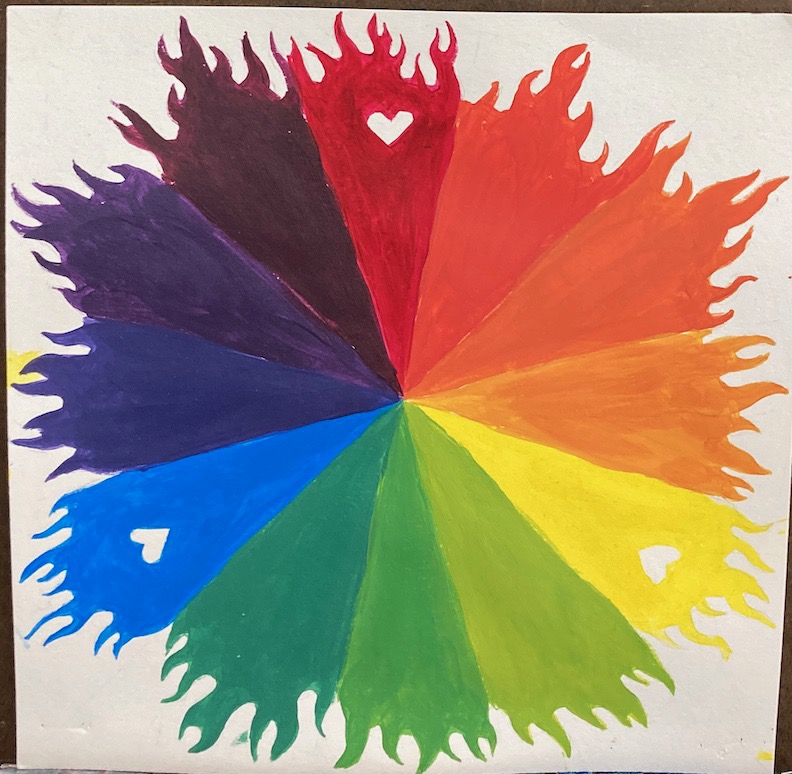This painting depicts a vibrant, circular emblem resembling a color wheel, segmented into pie-shaped wedges that radiate outward like flames. Set against a dark brown, textured background, the painting features twelve colors, arranged in the order of the rainbow. Starting from the top center (12 o'clock), a red wedge with a white heart is followed counter-clockwise by deep red, pink, brown, light blue, dark blue, green, light green, yellow with a white heart, bright orange, lighter orange-red, and bright orange-red. Each segment has corresponding flame-like extensions that maintain the same color, enhancing the dynamic, radiant appearance. The medium appears to be either acrylic paint or markers, with no text present anywhere on the image. Additionally, faint black outlines can be seen along the top left, right, and bottom edges, with a white streak in the lower left corner.